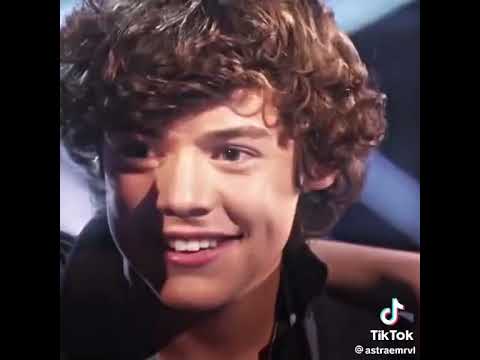The image is a screenshot of a young Caucasian man on TikTok, featuring his face from the neck up. He has a bright smile, showcasing his white top row of teeth, with his mouth slightly open. His head is tilted slightly downward and to the left. He sports thick, wavy brown hair, with long bangs that hang just below his left eyebrow, while the hair on the right side is parted to reveal his forehead above the right eyebrow. The young man has brown eyes, lightly tanned skin, and is wearing a black collared shirt. There's a shadow on the left side of his face, indicating the lighting is coming from the right. The TikTok logo is visible in the bottom right corner, along with the handle "Astromerville." The background features a black section on the left and right sides of the image, with a bluish-gray wall behind the man.